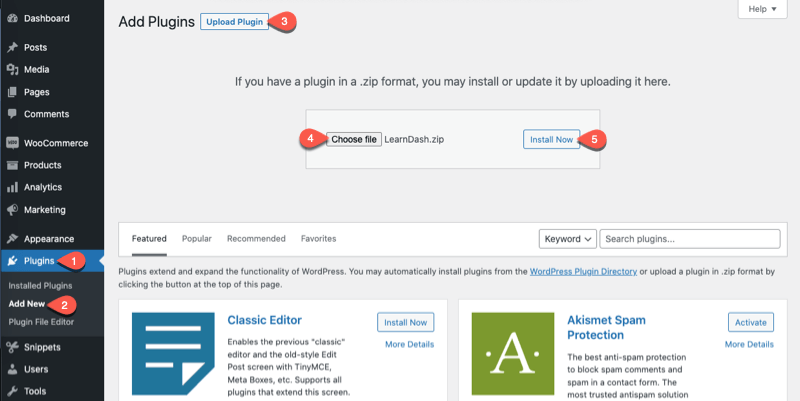The website screenshot displays a comprehensive guide on how to add plugins to WordPress. On the main section, located next to the "Add Plugins" header in white, there's a blue-button labeled "Upload Plugins" with a distinct blue outline. A red teardrop-shaped pin with the number 3 is visible, indicating an important notice.

In the gray instruction box, it states: "If you have a plugin in a .zip format, you may install or update it by uploading it here." Below that, there's a light gray file upload box displaying "learndash.zip" next to a "Choose File" button. Adjacent to this, there's an "Install Now" button in blue with a blue outline, accompanied by a number 5 in a red pin.

Further down, the number 4 pin in red points towards the "Choose File" button. In the upper right corner of the screen, there's a "Help" option with a dropdown menu. Below "Choose File," navigation tabs read "Featured," "Popular," "Recommended," and "Favorites," with the "Featured" tab underlined. A dropdown labeled "Keyword" and a search bar for plugins are also present.

Following this, a message in blue highlights that plugins enhance WordPress functionality and can be installed from the WordPress Plugin Directory or uploaded directly. Beneath this, two boxes feature plugins: "Classic Editor" and "Akismet Spam Protection," each with options to "Install Now" or "Activate" and a link for "More Details."

On the left sidebar, in a black section, various menu items are listed: "Dashboard," "Posts," "Media," "Pages," "Comments," "WooCommerce Products," "Analytics," "Marketing," "Appearance," and "Plugins," with a red pin numbered 1 next to "Plugins." The sub-menu under "Plugins" includes "Installed Plugins" with a red pin numbered 2, "Add New," "File Editor," and "Snippets." Additional items like "Users" and "Tools" are also shown.

Overall, the image provides a detailed walkthrough of the WordPress plugin installation process, complete with navigation indicators and functional descriptions.